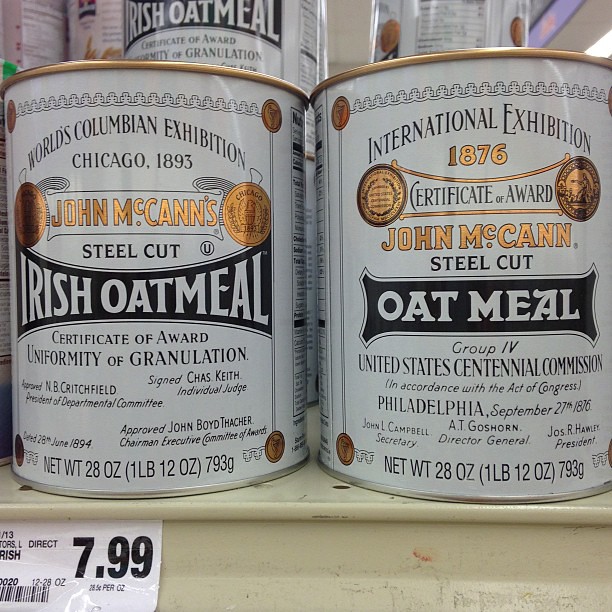The image depicts a close-up view of a store shelf displaying two prominently featured cans of oatmeal. Both cans have a white base with black text, accented by a decorative black border, and are capped with a gold lid. The can on the left bears the inscription "World Columbian Exhibition, Chicago, 1893" in bronze lettering at the top, followed by "John McCann's" encircled by two seals on either side. Below, it reads "Steel Cut Irish Oatmeal" and "Certificate of Award, Uniformity of Granulation."

To the right, a similar can showcases different text, stating "International Exhibition, 1876" at the top, alongside "Certificate of Award" and "John McCann" in bronze lettering. Further down, it highlights "Steel Cut Oatmeal, Group 4" followed by "United States Centennial Commission, in accordance with the Act of Congress, Philadelphia, September 27, 1876."

Both cans have identical dimensions and weight, noted as 28 ounces, 1 pound 12 ounces, or 793 grams. A price label below the cans indicates a retail price of $7.99. In the background, additional cans can be seen stacked, with one partially visible on the top left, bearing the label "Irish Oatmeal."